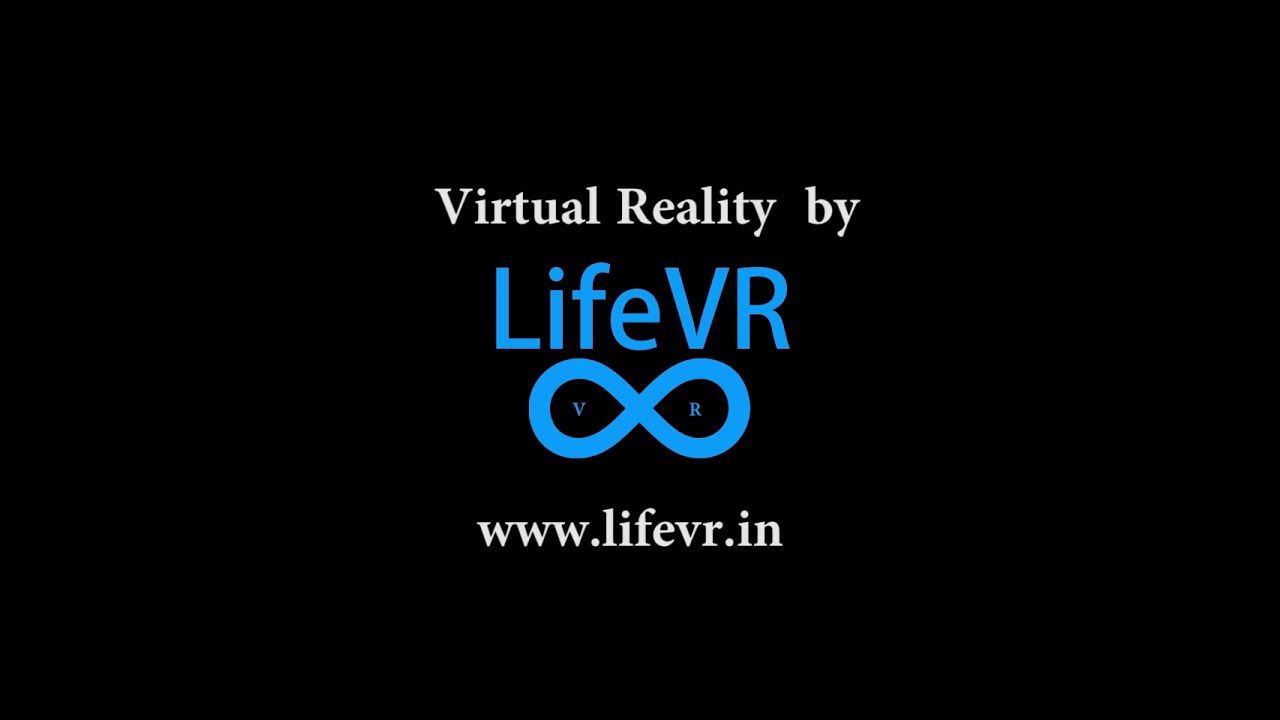The image features a black background with multiple lines of text and a logo centered prominently. At the top, white serif font reads "Virtual Reality by." Below this, large light blue uppercase letters spell out "Life VR." An infinity symbol colored in the same light blue lies underneath, with the letter "V" on the left circle and "R" on the right circle inside the symbol. At the bottom, white text displays the URL "www.lifevr.in." This image appears to be a promotional splash screen for Life VR, emphasizing the virtual reality theme.